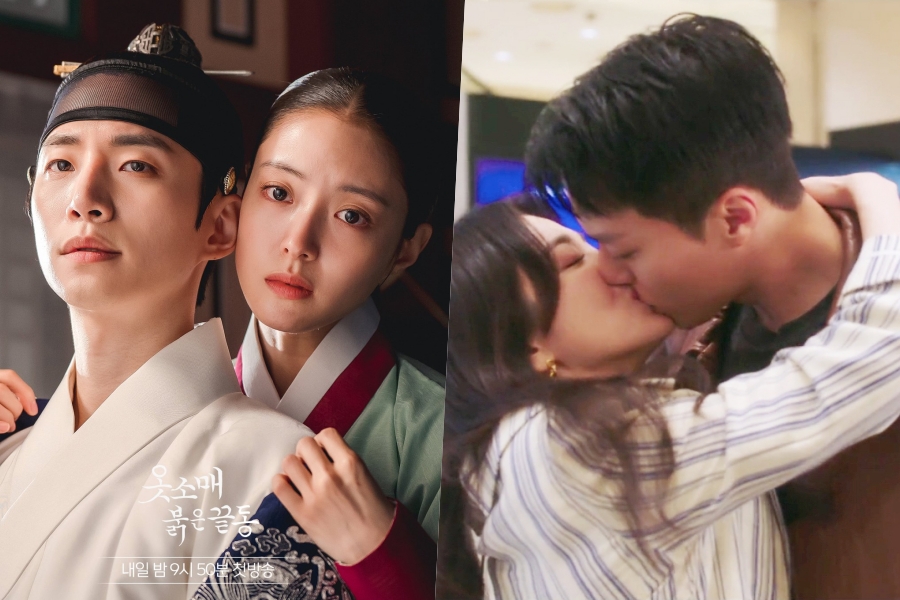This image consists of two distinct photographs side by side. In the left photograph, an Asian couple is dressed in traditional Korean attire, evoking the style of a historical drama or movie poster. The man wears a white kimono with blue designs on the sleeves and a black sheer cap featuring a metal structure. Standing behind him, the woman dons a green kimono with maroon and white edging; her black hair is slicked back and secured in a bun. She rests her hands on his shoulders. Korean text appears at the bottom of this image. The right photograph seems to depict the same couple in a modern setting, possibly at an airport. They are kissing, with the woman, who has long dark hair and is wearing a long-sleeved shirt, wrapping her arms around the neck of the man, who sports traditionally short hair and a brown shirt.